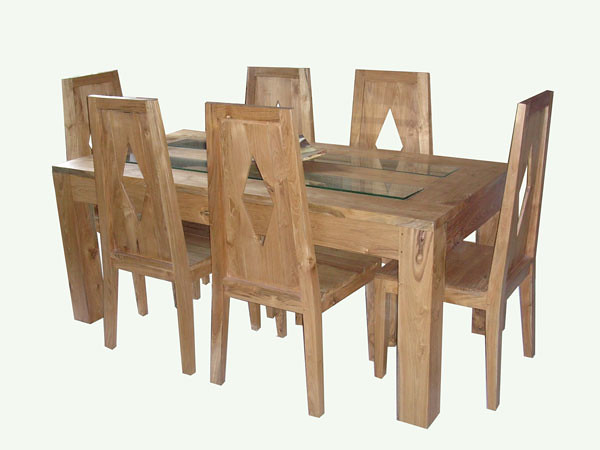This image showcases a beautifully crafted, light brown, solid wood dining table with a white or light blue background that is devoid of any additional elements, resembling a stock photo. The rectangular table features four large, robust rectangular legs and two clear, rectangular glass panes set into the center of the tabletop. Surrounding the table are six wooden chairs, arranged with one chair at each end and two on each of the longer sides. The chairs are meticulously designed with a diamond-shaped cutout in the middle of their rectangular backs, which taper from a wider base to a narrower top. The legs of the chairs are rectangular, ending in square bases where they meet the ground. The wood displays light tones with dark streaks, adding to the charm and elegance of the set. All chairs are neatly tucked into their respective spots around the table, enhancing the overall impression of order and sophistication.